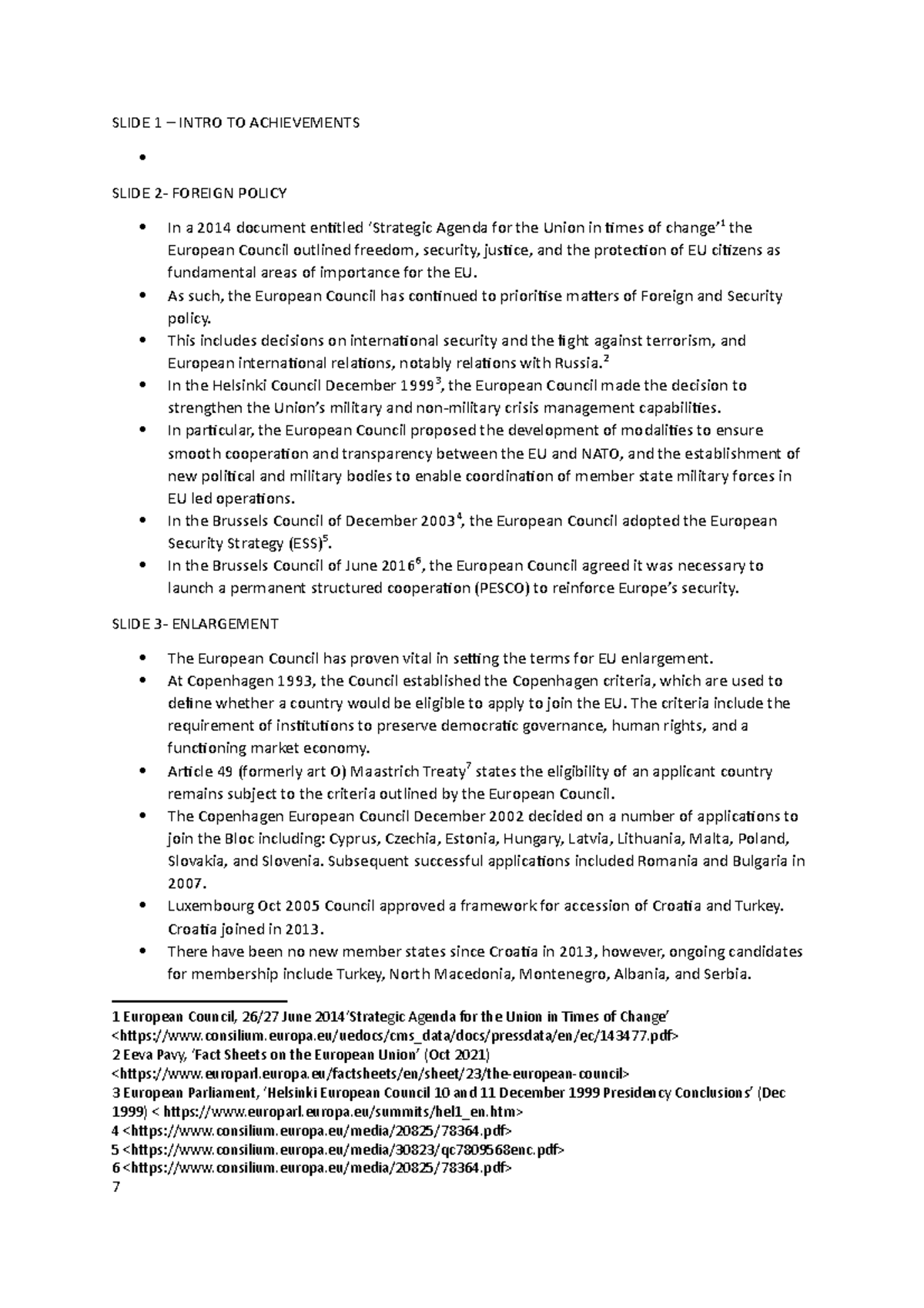The image is a screenshot of a text-based presentation containing black text on a white background. The content appears simple with plain lettering and no decorative elements. 

**Slide 1: Introduction to Achievements**
- The European Council penned a 2014 document titled "Strategic Agenda for the Union in Times of Change," highlighting freedom, security, justice, and the protection of EU citizens as core priorities.
- Consequently, the European Council has maintained a focus on foreign security and policy.

**Slide 2: Foreign Policy**
- The Council's agenda includes critical decisions on international security and combating terrorism, alongside European international relations, with notable emphasis on relations with Russia.
- There are additional points related to foreign policy following this.

**Slide 3: Enlargement**
- The European Council has played a crucial role in defining the terms for EU enlargement.
- At the Copenhagen summit in 1993, the Council established the Copenhagen Criteria, setting the standards for a country's eligibility to join the EU. These criteria require institutions that uphold democratic governance, human rights, and a functioning market economy.
- Article 49 is referenced, indicating continued elaboration on the enlargement criteria.

The bottom of the slide contains six footnotes, referencing the sources for the presented information.